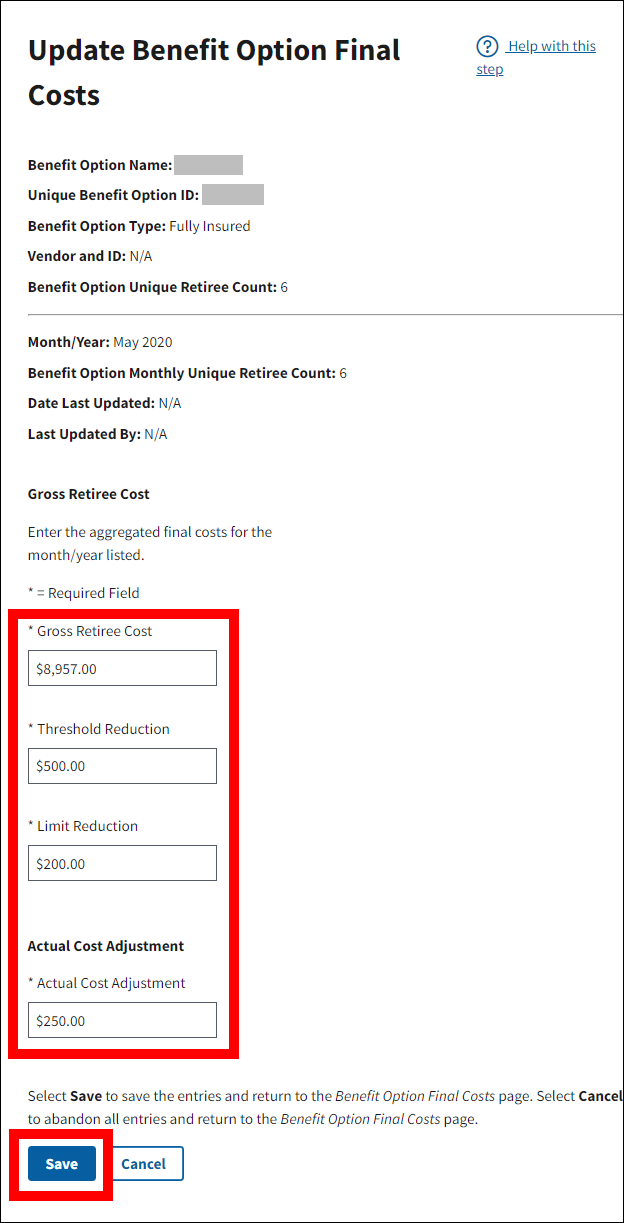The image showcases an electronic form titled "Update Benefit Option Final Costs." At the top right corner, there's a clickable link with a question mark icon labeled "Help with this step." Below this link are several fields and details:

1. **Benefit Option Name**: Redacted.
2. **Unique Benefit Option ID**: Redacted.
3. **Benefit Option Type**: Fully insured.
4. **Vendor ID**: N/A.
5. **Benefit Option Unique Retiree Count**: 6.
6. **Month/Year**: May 2020.
7. **Benefit Option Monthly Unique Retiree Count**: 6.
8. **Date Last Updated**: None.
9. **Last Updated By**: None.
10. **Gross Retiree Cost**: Contains a dropdown to enter the aggregated final cost for the listed month, marked as a required field with an asterisk.

There are four required input boxes below this section:
- **Gross Retiree Cost**: Approximately $9,000.
- **Threshold Reduction**: $500.
- **Limited Reduction**: $200.
- **Actual Cost Adjustment**: $250.

At the bottom of the form, there are "Save" and "Cancel" buttons.